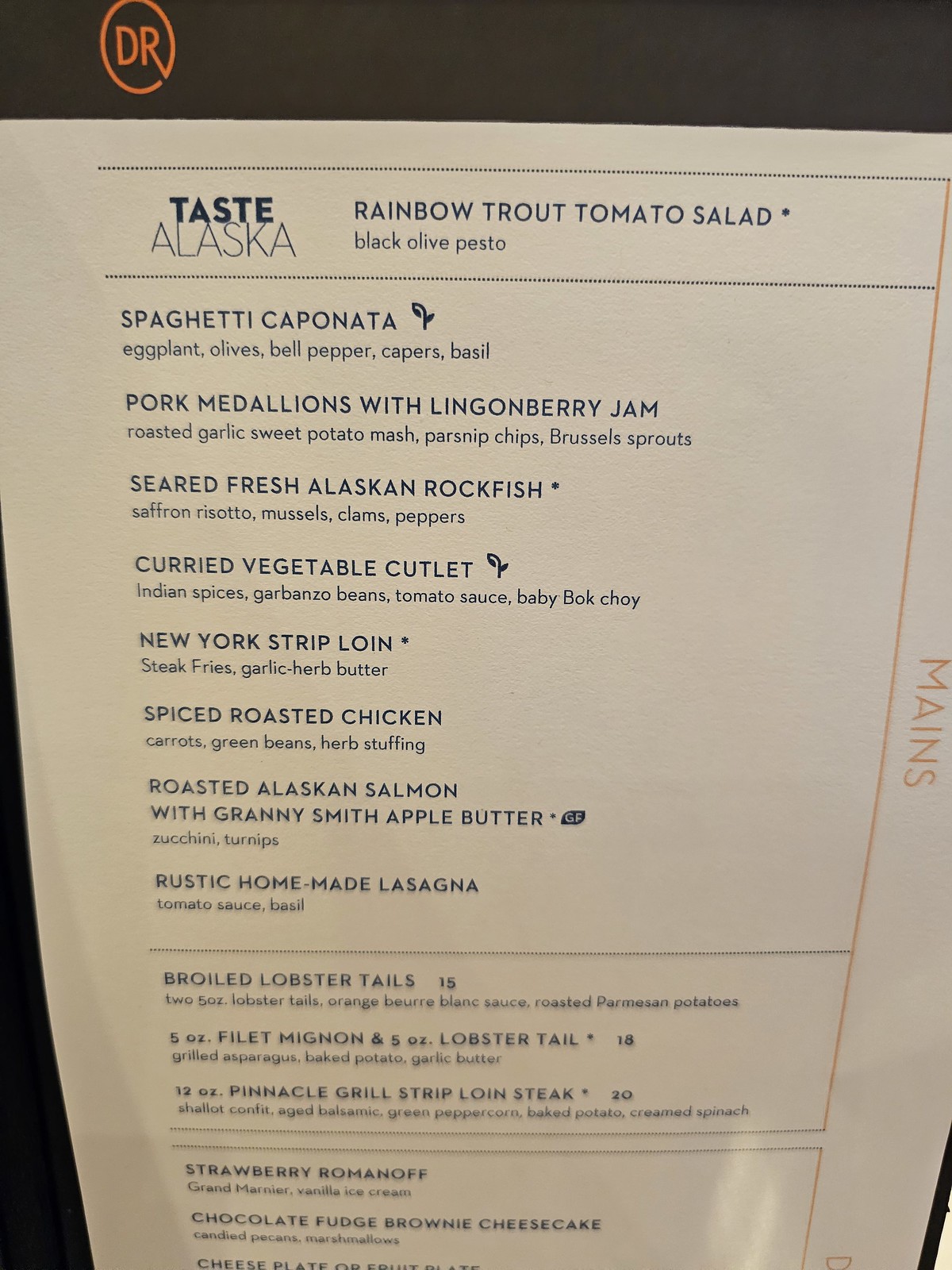This is a detailed color photograph of a menu titled "Taste Alaska" in blue at the top. The menu's offerings are divided into sections, starting with appetizers which include "Rainbow Trout Tomato Salad" served with Black Olive Pesto. The main courses are as follows:

- "Spaghetti Caponata" which consists of eggplant, olives, bell pepper, capers, and basil.
  
- "Pork Medallions" served with lingonberry jam, roasted garlic, sweet potato mash, parsnip chips, and Brussels sprouts.
  
- "Seared Fresh Alaskan Rockfish" which is accompanied by saffron risotto, mussels, clams, and peppers.
  
- "Curried Vegetable Cutlet" made with Indian spices, garbanzo beans, tomato sauce, and baby bok choy.
  
- "New York Strip Loin" served with steak fries and garlic herb butter.
  
- "Spiced Roasted Chicken" paired with carrots, green beans, and herb stuffing.
  
- "Roasted Alaskan Salmon" finished with a Granny Smith apple butter.